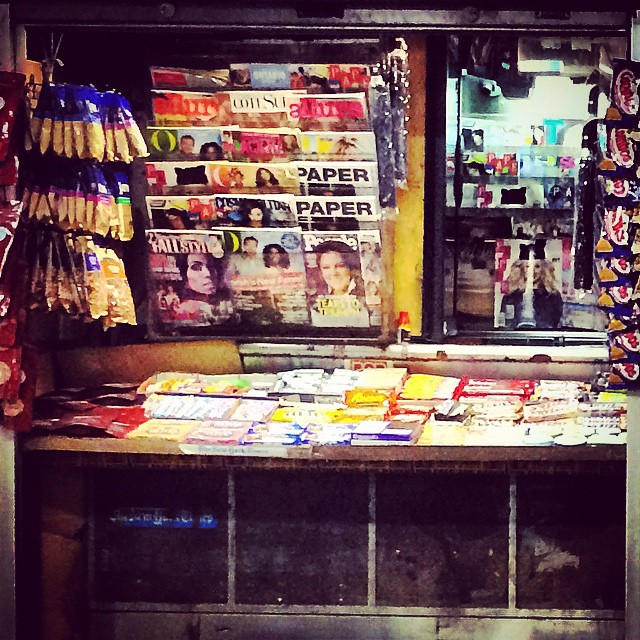The photograph depicts a vintage sidewalk newsstand from the 1960s or 1970s, reminiscent of those seen in Times Square, New York. The newsstand, constructed from shabby gray wood with brown planks, features a distinct cutout window for the absent clerk. The back wall, painted in red and yellow, prominently displays a rack holding three columns of magazines, each column containing six magazines. Notable titles include 'People' and 'Allure,' among others. To the left of the clerk's window, individual snack servings such as peanuts and cashews hang from hooks. Beneath these snacks, a shelf runs horizontally, stocked with boxes of gum and mints. On the right side, there are hanging chips and a red and black item, along with a black-trimmed mirror affixed to the back wall. A table in front of the counter is spread with various maps and literature, adding to the eclectic assortment of items. The faded photograph also hints at miscellaneous knickknacks and a picture of a woman in the background, evoking a nostalgic, crowded charm.